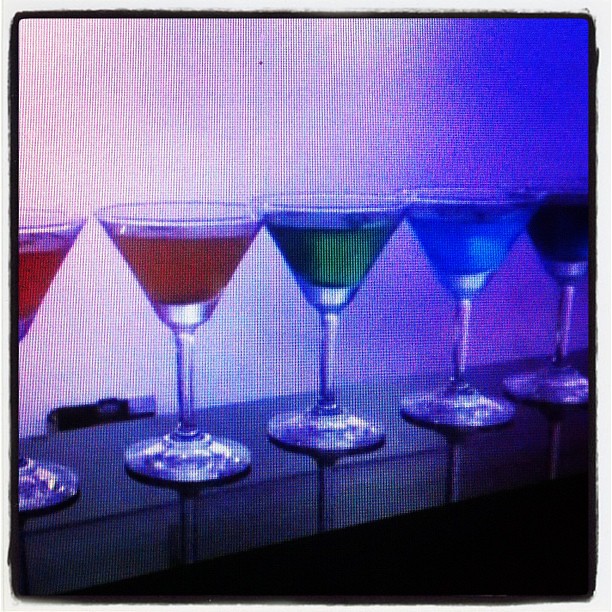This image is a photograph of five martini glasses arranged horizontally on a gray countertop against a white wall. Each glass contains a differently colored liquid: the first two glasses have a red liquid, the third has green, the fourth has light blue, and the fifth has a dark, nearly black liquid. The photograph has a unique, vintage filter, making it appear as if it's being viewed through a mesh screen or an old CRT television, with a purple, pixelated overlay. Additionally, there is a black border around the image, with an outer white paper border, suggesting that the photograph might be a picture of a printout.